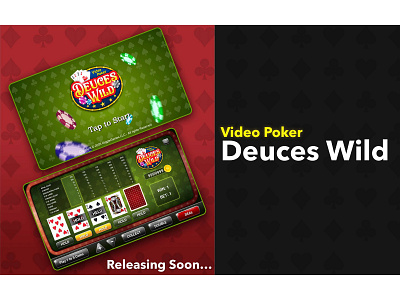The image portrays an advertisement for a video poker game titled "Deuces Wild." It features a two-toned background with the left side showcasing a maroon color adorned with card suits—clubs, spades, and diamonds—and the right side in black. On the black background, the text "Video Poker" in bold yellow letters and "Deuces Wild" in white are prominently displayed. 

On the maroon side, there are two distinct rectangles. The top rectangle features the game's logo, characterized by orange lettering on a blue background, and contains a green box with the words "Deuces Wild" along with a prompt to "Tap to Start." Below this, there's another box indicating the game is "Releasing Soon," accompanied by an image of poker chips seemingly in mid-toss.

The entire design suggests that the game, which seems to be accessed via a computer, is engaging and user-friendly, poised to launch soon. The lid of the tin box in the image also reflects the same text and design cues, further tying in the overall theme of the game.